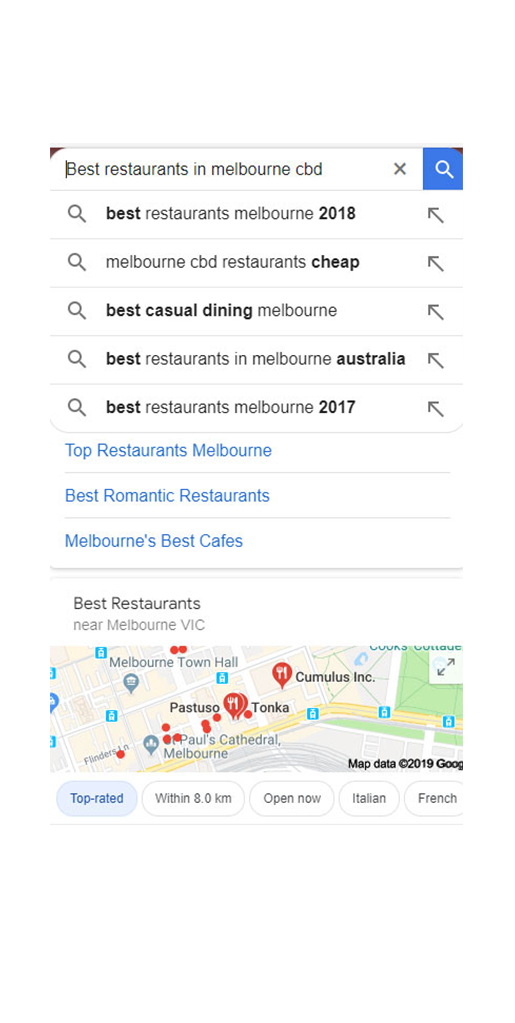Close-up image of a Google search results page. The search box at the top center is prominently displayed with a query typed in black text: "Best restaurants in Melbourne CBD." The corners of the search box are tinted red on both the left and right sides. The search box's main section is white, transitioning to blue on the right side where there is a white magnifying glass icon superimposed. 

Below the search box, various search result suggestions are listed. Each suggestion is preceded by a black magnifying glass icon and various shades of text:

1. "Best restaurants in Melbourne 2018"
2. "Melbourne CBD restaurant guide"
3. "Best casual dining in Melbourne"
4. "Best restaurants in Melbourne, Australia"
5. "Best restaurants Melbourne 2017"
6. In blue text: "Best restaurants Melbourne"
7. A gray dividing line
8. In blue text: "Melbourne's best cafe"
9. A gray dividing line
10. In black text: "best restaurants Melbourne"

Below the list of suggestions, a map is partially visible with highlighted locations, including "Patuxo," "Taco," and "Blackstone," which are marked as some of the best restaurants.